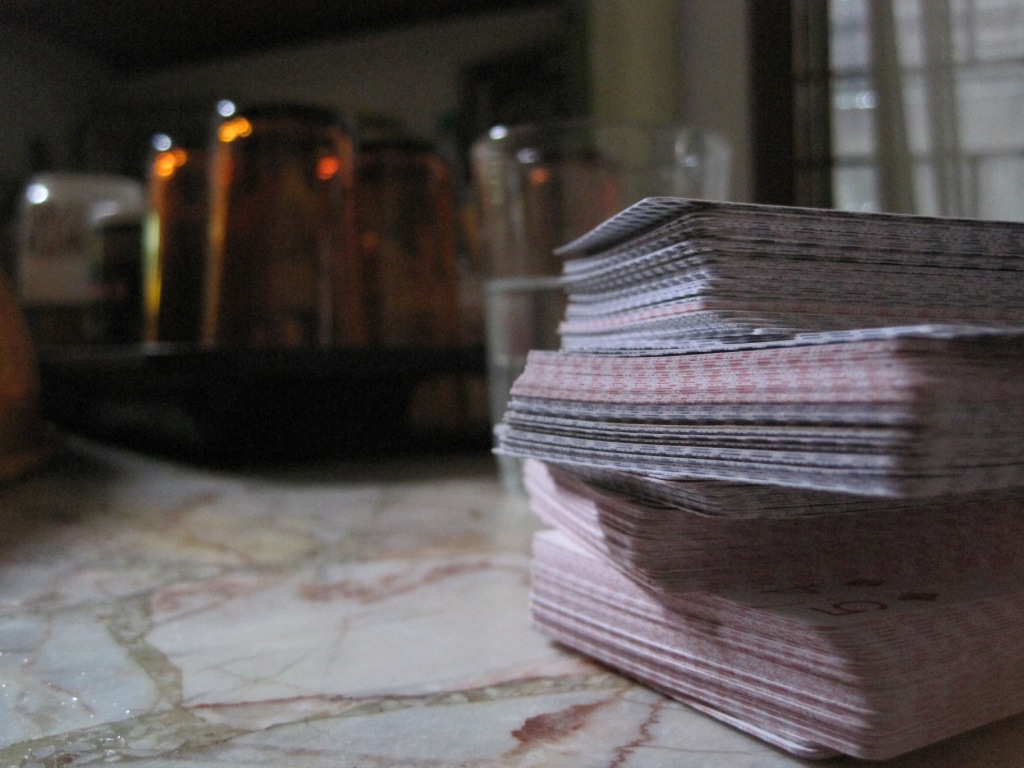The photograph showcases a meticulously arranged stack of playing cards prominently situated in the front right corner of the frame. Multiple decks are present, each varying slightly in color and pattern. The top deck features a red and white border with the five of diamonds clearly visible at the top. Beside it, a second deck combines red, white, and blue elements and is slightly angled to the left. Positioned next, another stack leans back to the right, featuring mainly blue and white cards with a few red and white ones on top. Further to the left, an almost entirely blue and white stack with sporadic red and white cards completes the arrangement. 

The playing cards rest on a granite-style countertop characterized by an off-white base with intricate gray and red veining. Slightly back from the card stacks, a glass filled halfway with water is placed, adding a touch of simplicity to the scene. In the background, a black tray is visible, holding three upside-down brown glasses. Beyond this, a window fitted with a gray curtain is faintly discernible, contributing to the slightly blurred and out-of-focus backdrop that provides depth to the image.